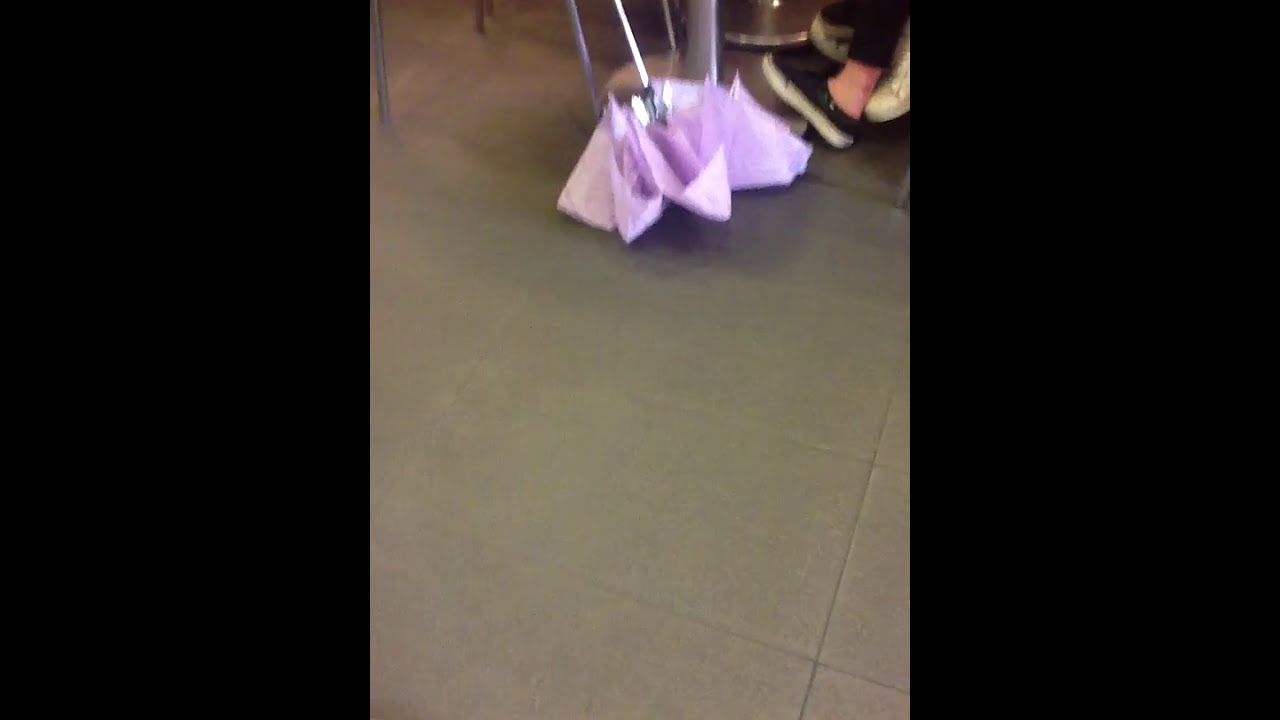In this photograph, the ground is made of square-shaped grey tiles arranged in a grid pattern. Dominating the top section of the image is a light lavender umbrella lying on the floor, which some might mistake for bags or purses. Behind the umbrella, there is a metallic silver pole, likely a table leg, accompanied by a couple of thinner poles nearby. To the right of the umbrella, a foot is visible, revealing a white-skinned ankle and lower leg, covered by a black slip-on shoe with a white tread. The top portion also includes what appears to be a table with a circular base, similar to what one might see in a restaurant, with chairs pulled up to it. The sides of the image are framed by two vertical black strips.